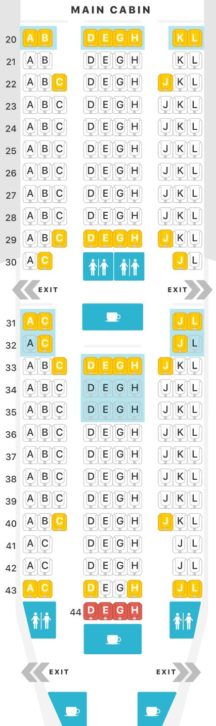The image shows the intricate seating arrangements inside a cabin with seats numbered along the left-hand side from 20 to 43. The majority of the seats are grey, while others are highlighted in orange, red, and light blue. Here is the detailed breakdown of the seat colors:

- Row 20: Seats A, B, D, E, G, H, K, and L are both orange and blue.
- Row 22: Seats C and J are orange.
- Row 29: Seats C, D, E, G, H, and J are orange.
- Row 30: Seats C and J are orange.
- Row 31: Seats A, C, J, and L are both orange and blue.
- Row 32: Seats C and J are both orange and blue.
- Row 33: Seats C, D, E, G, H, and J are orange, while seats D, E, G, and H are also blue.
- Row 34: Seats D, E, G, and H are light blue.
- Row 35: Seats D, E, G, and H are light blue.
- Row 40: Seats C and J are orange.
- Row 43: Seats A, C, D, H, J, and L are orange.
- Row 44: Seats D, E, G, and H are red.

This arrangement highlights a striking pattern of colour-coded seating within the cabin.